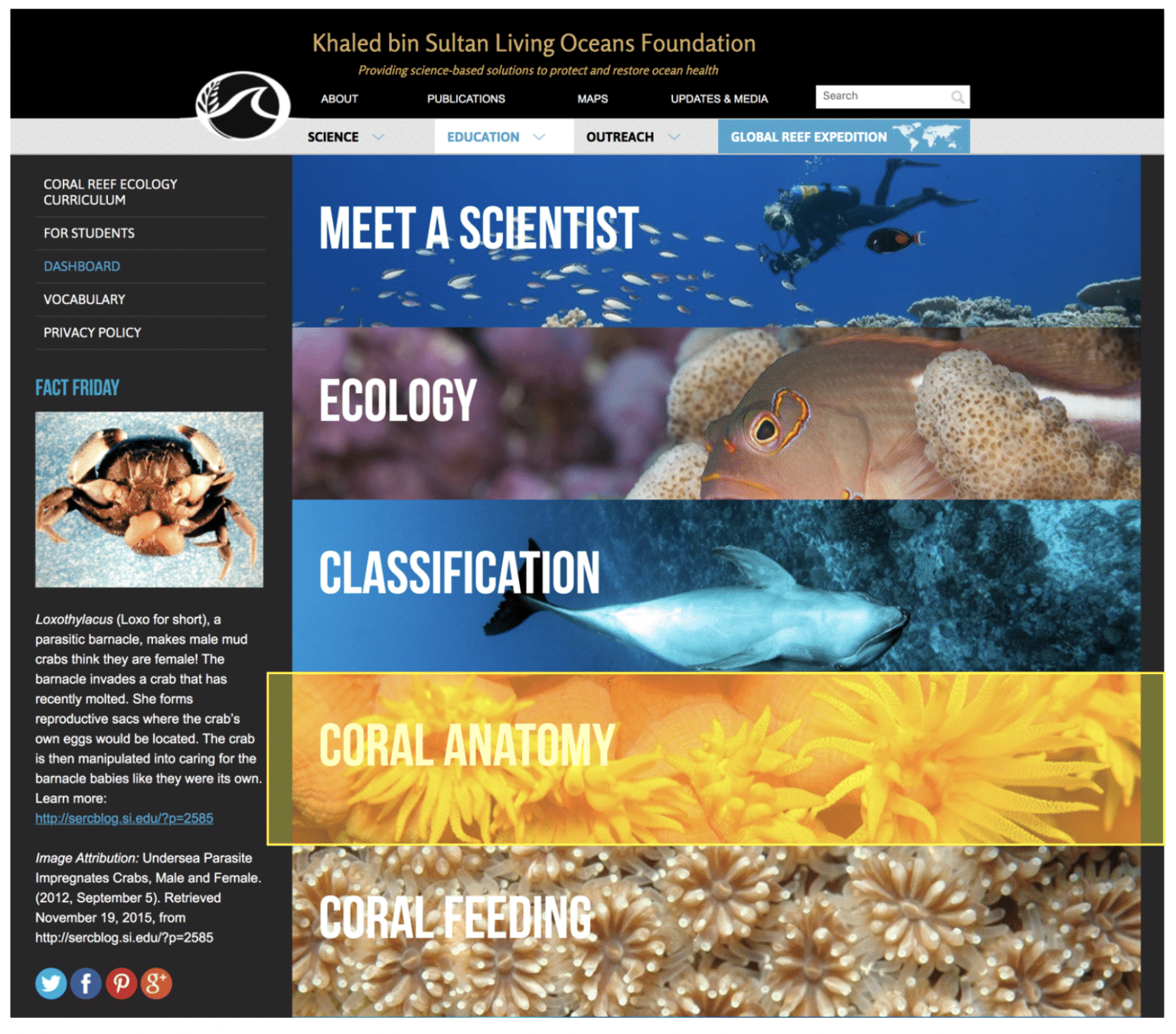This image features a prominently displayed horizontal banner stretching from left to right. The banner consists of a black bar in the middle, holding a goldish-yellow font that reads: "Khaled bin Sultan Living Oceans Foundation." Below this, in a smaller font, it states: "Providing science-based solutions to protect and restore ocean health."

Beneath the banner, there are five distinctive blocks arranged horizontally. 

1. The first block, labeled "Meet a Scientist," displays an image of a person scuba diving.
2. The second block, titled "Ecology," showcases a close-up photograph of fish underwater.
3. The third block, named "Classification," features a striking image of a dolphin swimming upside down underwater.
4. The fourth block, called "Coral Anatomy," stands out with a yellow border and depicts what appears to be flowers in the background.
5. The final block, "Coral Feeding," presents an image of a vibrant coral reef.

Additionally, there is a vertical menu located on the left side of the image, providing further navigation options.